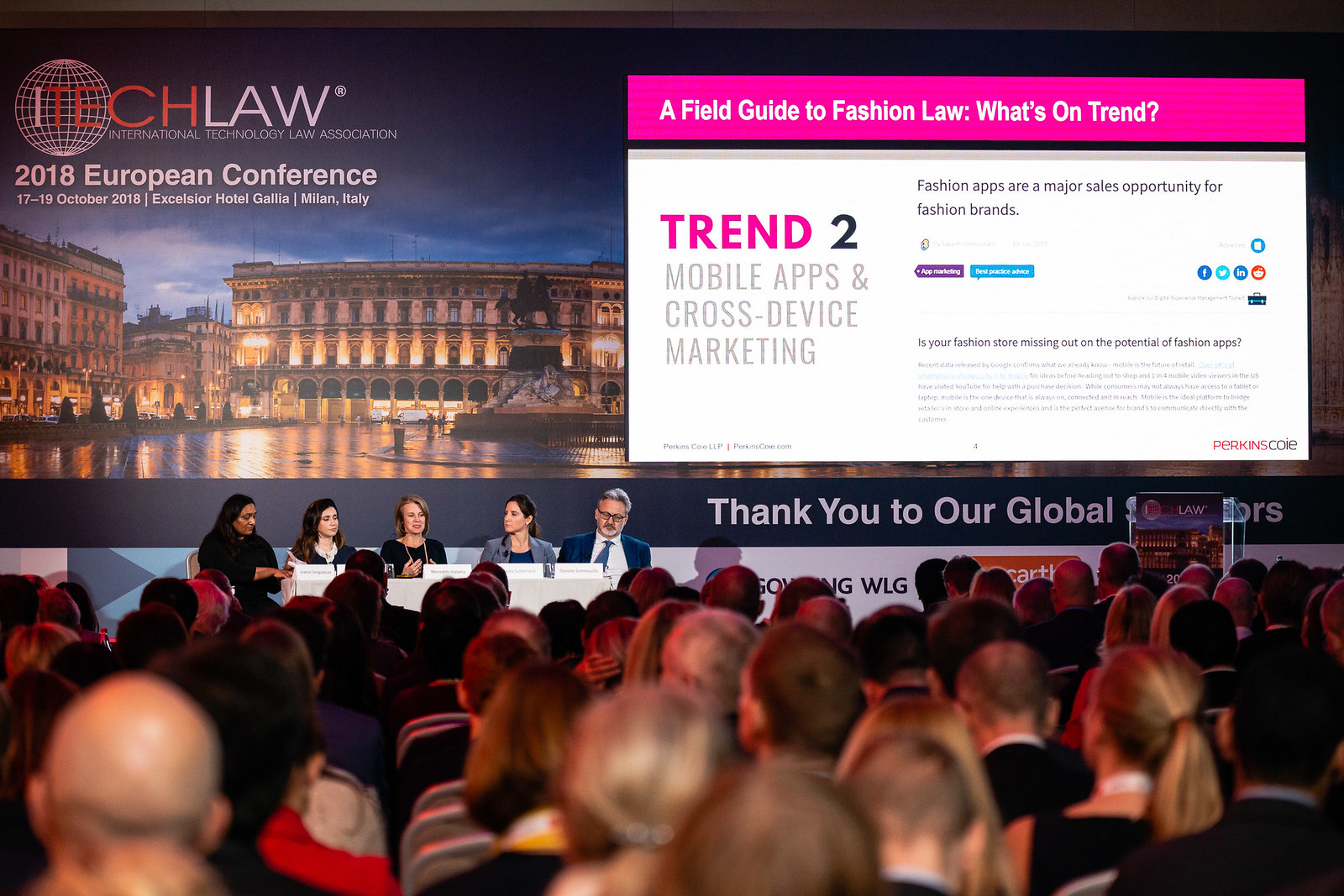This photo captures a session at the International Technology Law Association's (ITECH Law) 2018 European Conference, held at the Excelsior Hotel Gallia in Milan, Italy, from October 17 to 19, 2018. The image is taken from the perspective of an audience member, showcasing a large crowd of approximately 50 people seated and facing a stage. On the stage, there are five panelists—four women and one man—sitting behind a white table with name cards in front of them. The background features a large projection screen displaying the conference title and location details. The screen also highlights the panel's discussion topic: "A Field Guide to Fashion Law: What's On Trend" with a focus on mobile apps and cross-device marketing. Additionally, the screen mentions fashion apps as a major sales opportunity for fashion brands and includes options for liking and sharing recommendations. This detailed setting reflects the importance and international scope of the conference, with attendees deeply engaged in the presentation.